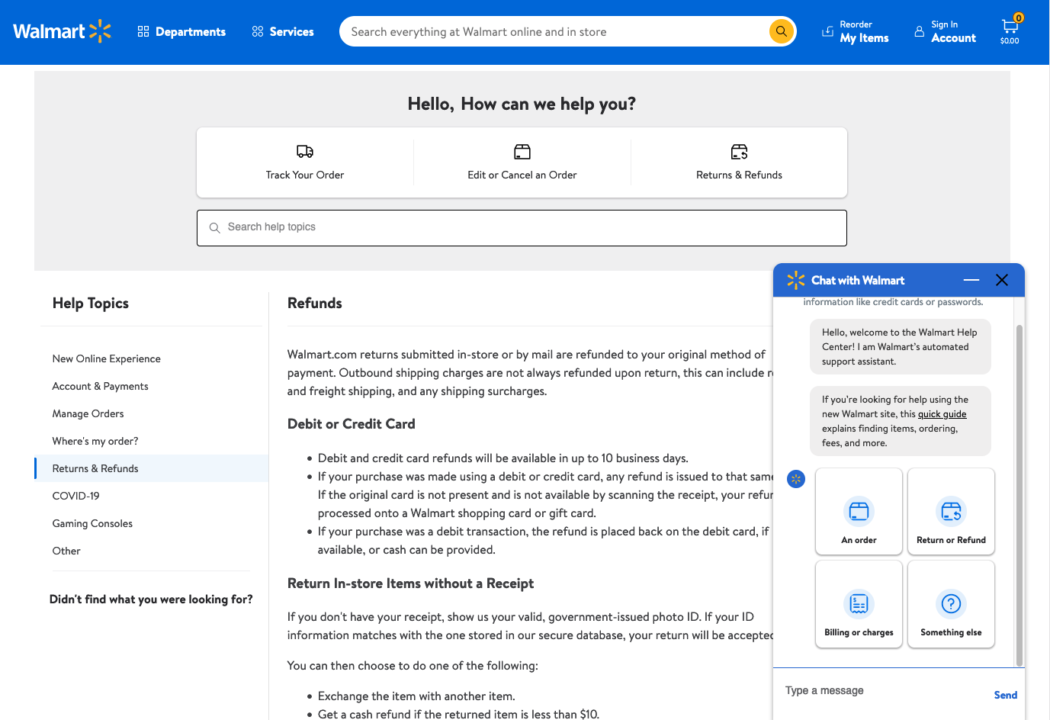This image is a detailed screenshot of Walmart's customer support webpage. At the top of the page, the header is dominated by Walmart’s signature bright blue color, featuring the iconic yellow Walmart logo on the left. Adjacent to the logo, there are links for “Reorder My Items,” “Sign In,” and a shopping cart icon displaying zero items.

On the left-hand side of the page, a navigational sidebar lists various help topics, with "Returns and Refunds" currently selected. The help topics menu includes options for "New Online Experience," "Account and Payments," "Manage Orders," "Where’s My Order," "Returns and Refunds," "COVID-19," "Gaming Consoles," and "Other." At the very bottom of this list, there is an option labeled "Didn't find what you were looking for?"

Centered on the page, a prominent search bar invites users with the message: "Hello, how can we help you?" Below this, there are quick-links for common inquiries such as "Track Your Order," "Edit or Cancel an Order," and "Returns and Refunds."

In the main content area, detailed information about returns and refunds is displayed. Subsections here include guidance on "Returning and Store Items without a Receipt" and information regarding "Debit or Credit Card" refunds. 

At the bottom of the content is a text box open for chatting with Walmart support, initiated by a chatbot. However, no user message has yet been entered in this conversation. 

All these elements combined create an intuitive and organized layout designed to assist users in resolving their inquiries efficiently.